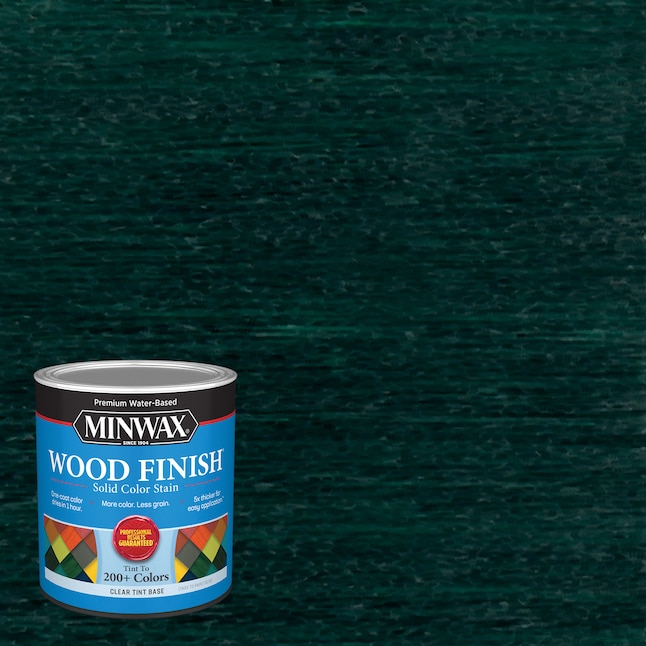The image depicts a detailed advertisement for Minwax's premium water-based wood finish solid color stain. The background of the image is an intricate, emerald, dark green texture with streaks of white, resembling a static-y green television screen. This textured background covers about three-fourths of the image, leaving the bottom fourth largely empty except for a prominently featured Minwax paint can in the bottom left corner. 

The can itself is a cylinder with a silver metal lid and a black band across the top. On this black band, in white text, are the words "premium water-based." Below this are the Minwax logo and the product name in white over a blue background: "wood finish, solid color stain." Additional text on the can touts features such as "one coat color, dries in one hour, more color, less grain, so thick for easy application." A red circle with yellow text suggests some sort of guarantee. Further details include "tint to 200+ colors" and "clear tint base" written in black text against a white strip. The label is complemented by a crosshatch of multicolored squares to visually represent the variety of colors available for tinting, including hues like orange, yellow, green, and gray. The rest of the picture remains a stark, uninterrupted green backdrop, emphasizing the can as the central focus.